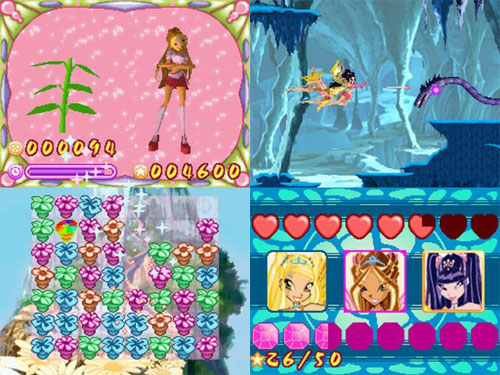The composite image, divided into four equal sections, presents a colorful and dynamic anime-themed scene. 

In the upper left section, set against a predominantly pink background, stands a character with elongated legs, adorned in a pink shirt, red skirt, tall white socks, and red shoes. To her right is a small green plant, with a yellow number "000094" written below.

The upper right section depicts an intense scene where three female characters with various hair colors are flying toward a blue snake-like creature inside an ice cave. The characters are shooting pink cannons, and the cave environment is depicted with dark blue water and an icy, bluish cavern.

The bottom left section appears to be a puzzle game interface featuring vividly colored tiles resembling flowers. The scene is divided by lines that resemble a sliding puzzle game, with flower tiles in green, pink, and blue hues.

The bottom right section showcases three female anime characters: one with pink and blue hair, one with brown hair, and one blonde with a yellow framed backdrop. Above their heads are hearts—red hearts on the left and brown hearts on the right, with one slightly cut off at the top. Below the characters are pink crystals, one of which is half-formed, and a score of "26/50" highlighted in yellow.

Combining elements from all sections, the image blends vibrant characters, dynamic action scenes, and game elements into a cohesive and engaging visual experience.